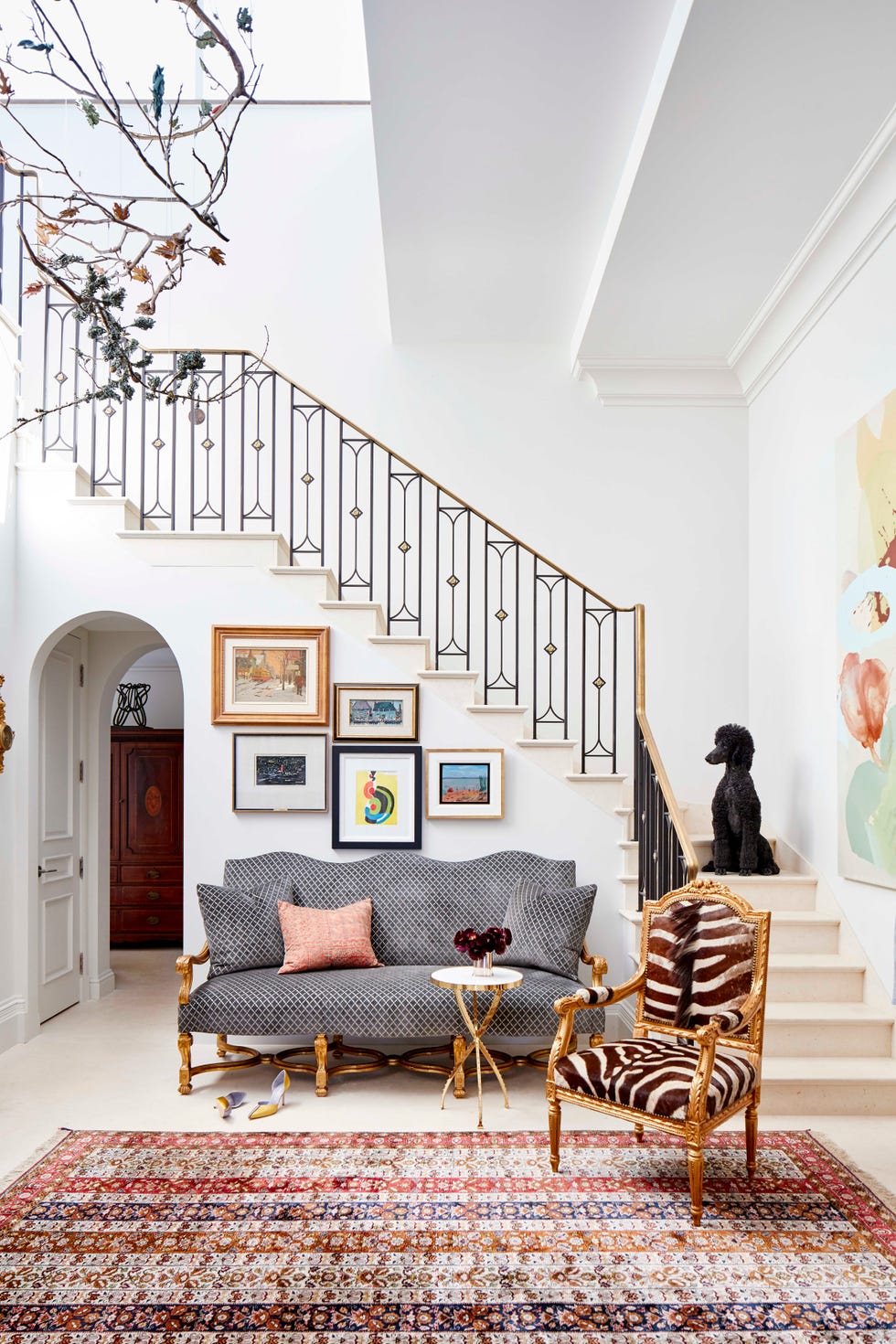The image depicts a bright living room characterized by white walls and a striking staircase leading to the upper floor with gold and black wrought iron railings. Dominating the floor is a richly patterned Turkish rug in hues of red, blue, gold, and white. At the bottom of the steps sits a luxurious zebra-print armchair with gilded gold accents. Adjacent to the armchair, on the rug, stands a dark gray and white checkered couch adorned with various throw pillows, including a notable pink one. In front of the couch, a white side table with gold legs displays a vase of fresh flowers.

The living room features a collage of pictures on the wall, contributing to the cozy and personalized atmosphere. Just by the couch, a pair of high heels is casually tossed to the side. Adding to the room's elegance is a black standard poodle perched about five or six steps up the staircase, surveying the space.

To the far right, a doorway with arched trim reveals a glimpse of another room potentially housing a dark mahogany armoire. Suspended from the ceiling near the top of the image are branches or plant leaves, possibly from a large vase or planter situated above. Completing the scene is an abstract floral painting mounted on the wall by the stairs, adding a final touch of artistry to this detailed and luxurious living room setup.